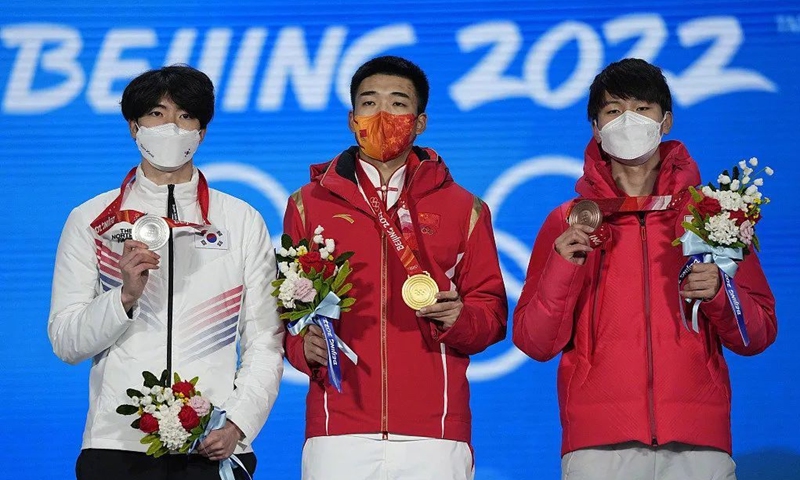In this live photograph from the Beijing 2022 Olympics, three Asian male athletes are standing in a row against a backdrop featuring the event's title and Olympic symbol, which are set against a gradient of light to darker blue. All three are wearing COVID masks and are standing close together, highlighting camaraderie despite the necessary precautions.

The athlete on the left is dressed in a white long-sleeved shirt and black pants. His white mask complements his attire, and he proudly holds up a silver medal in his right hand and a bouquet of flowers adorned with white and red blooms, green leaves, and a blue ribbon in his left. His short black hair is neatly styled.

In the center, the gold medalist stands out in a striking red jacket paired with cream and white pants and a red and yellow-orange mask. He is also holding a bouquet of similar flowers in his right hand while displaying his gold medal prominently. His short black hair retains a neat and tidy appearance.

On the right, the bronze medalist is clad in a thick red "marshmallow" coat, also with cream and white pants. His white mask matches that of the athlete on the left. He holds his bronze medal in his left hand and a matching bouquet of flowers in his right. Like his fellow athletes, his short black hair is neatly styled.

The image captures a significant moment of triumph and unity among these athletes, their expressions muted by their masks but their achievements clear in the medals they proudly display.